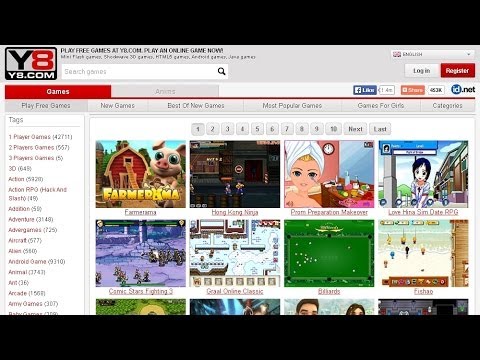Screenshot of Y8.com Homepage

The screenshot is a horizontal capture of the Y8.com homepage, a platform known for offering free online games. The topmost section displays a black navigation bar, immediately followed by the site's logo. The logo comprises the letters "Y8" within a square—"Y" being black and "8" colored red. Adjacent to the logo, the text "Y8.com" is prominently displayed, followed by the slogan, "Play free games at Y8.com. Play an online game now," mostly aligned to the left-hand side.

Underneath the logo and slogan, a red menu button labeled "Games" is visible. To its right, there is another menu button, though the text is greyed out and unreadable. The rest of the menu extends horizontally, featuring options such as "Play Free Games," "New Games," "Best of New Games," "Most Popular Games," "Games for Girls," and a "Categories" button at the far right.

Beneath this primary menu bar, the main content area showcases a grid of eight colorful game thumbnails. Each thumbnail provides a visual snippet of the game it represents, adorned with cartoonish characters and vibrant designs. Notable game titles include "Farm America" and "Hong Kong Ninja."

At the very bottom of the screenshot, there's a black band marking the end of the visible page.

This detailed layout provides a clear view into the structure and design of the Y8.com homepage, emphasizing its focus on easy navigation and an array of gaming options.